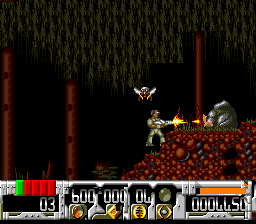A screenshot from a retro-style video game depicts a scene set against a predominantly black background. The environment features three brown cylindrical shapes resembling tree trunks, draped with green, vine-like leaves. In the foreground, a character dressed in green wielding a silver gun is visible, with an orange explosion emanating from the weapon as it fires bullets toward a gray-colored rock. The ground beneath the character is textured with red rocky patterns. Positioned in the bottom left corner, a health bar displays one green block followed by four red blocks, alongside text indicating "03" and "600000." Additionally, the score is highlighted, reading "0004450."